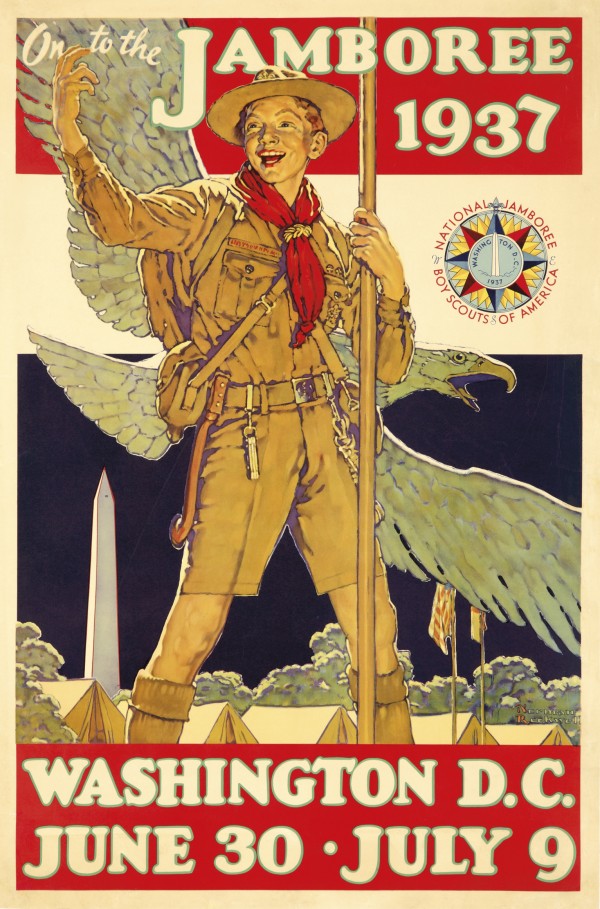This vintage poster advertises the 1937 National Jamboree for the Boy Scouts of America, held in Washington, D.C., from June 30th to July 9th. Dominating the center is an image of a young Boy Scout dressed in a classic tan uniform with long tan socks and a red scarf, topped with a wide-brimmed hat. He holds a long wooden walking stick in his left hand while his right hand is raised as if welcoming or exclaiming something. Behind him, an eagle soars with its wings outstretched. At his feet are teepees and forested scenery, adding to the adventurous ambiance of the scene. The top of the poster features bold white text on a red backdrop that reads, "On to the Jamboree, 1937," while the bottom bears the event's details: "Washington, D.C., June 30th to July 9th." To the right, a red, yellow, and black medallion with a star and the image of the Pentagon reads, "National Jamboree, Boy Scouts of America." The colors of the poster, including faded hues of red, cream, khaki, and green, reinforce its vintage appeal.